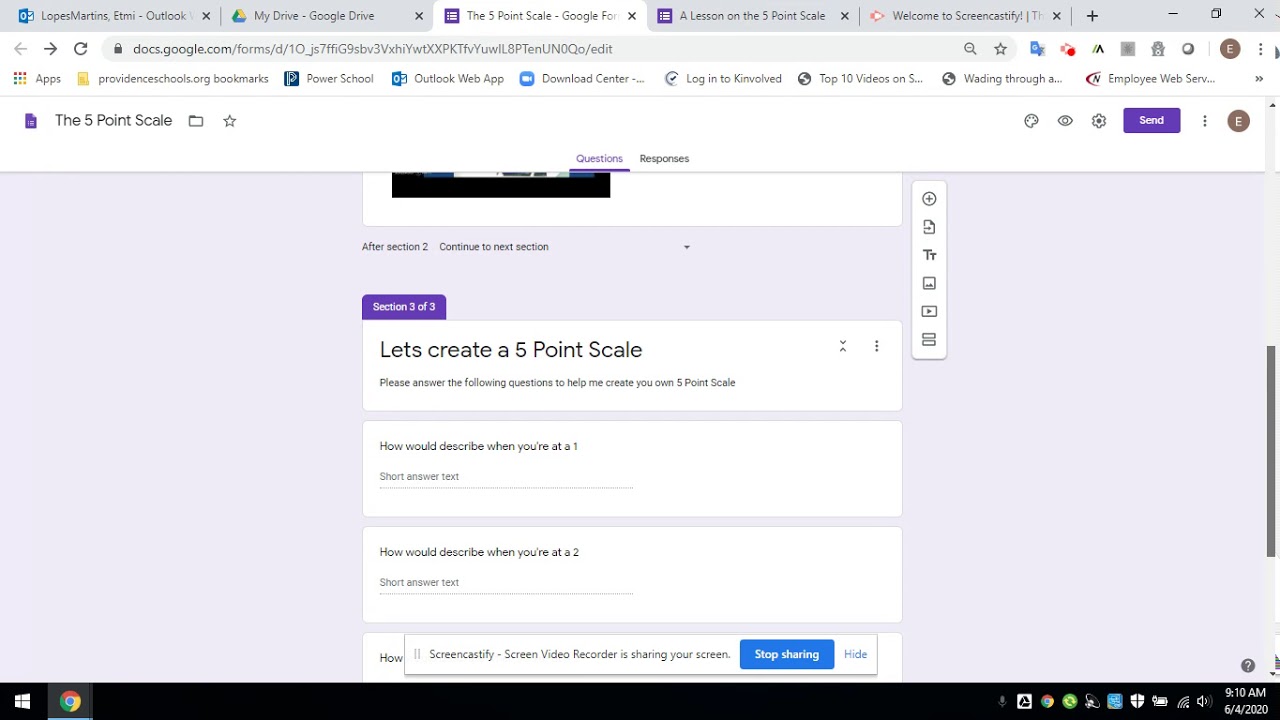A screenshot of a computer screen displaying multiple browser tabs is featured. The tabs span across the top of the screen and include the following titles: "Lopez Martinez," "Outlook," "My Drive - Google Drive," and the currently open tab, "Five-Point Scale - Google Forms." To the right, additional tabs include "Lesson on Five-Point Scale" and "Welcome to Screen Certify." The open tab indicates that the user is engaged in learning how to utilize a five-point scale via Google Forms.

Beneath the browser tabs, the URL bar and various navigation buttons, including a 'forward' button, are visible. There is also an options icon resembling a small cube, which, when clicked, reveals additional application choices such as "ProvidenceSchools.org," "Bookmarks," "PowerSchool," "Outlook Web," and the "Download Center." Other accessible options include "Log on to Kenvolve" and "Top Ten Videos."

The user has opened the "Five-Point Scale" form and is currently navigating section three of three, which prompts the creation of a personalized five-point scale. It requests users to answer a series of questions to complete the scale creation process. The interface suggests that upon finishing, users can select a 'stop sharing' button, indicating this may be part of a screencast visible to others, potentially for educational purposes.